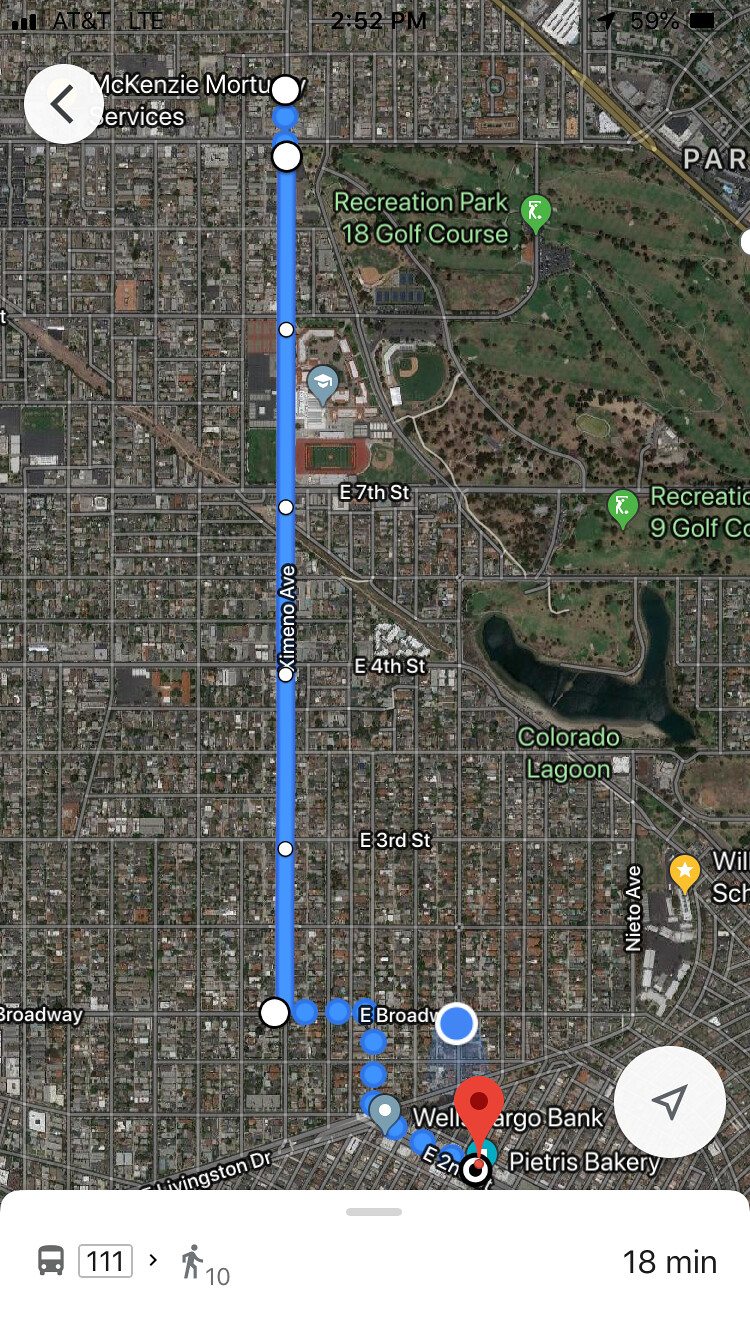The image depicts a satellite view of a map with a detailed navigation route. Dominating the map is a prominent light blue vertical line with multiple interspersed white dots, indicating key points along the route. Connected to this main vertical line are smaller blue and light blue lines branching off to the right, leading to a notable white dot with a black center, complemented by a red location arrow indicating the current position of the user. 

In the upper right corner, a green-colored area is labeled "Recreation Park 18 Golf Course." Just below this green area lies a U-shaped body of water named "Colorado Lagoon," displayed in green letters.

At the top of the light blue vertical line, there is white text indicating "McKinsey Mortuary Services." 

Below the map, there are icons and numerical details providing additional information: a bus symbol with the number 111, a walking man symbol with the number 10, and an indication of "18 minutes" on the lower right side. The map is otherwise devoid of additional text, focusing solely on the aforementioned locations and navigation aids.